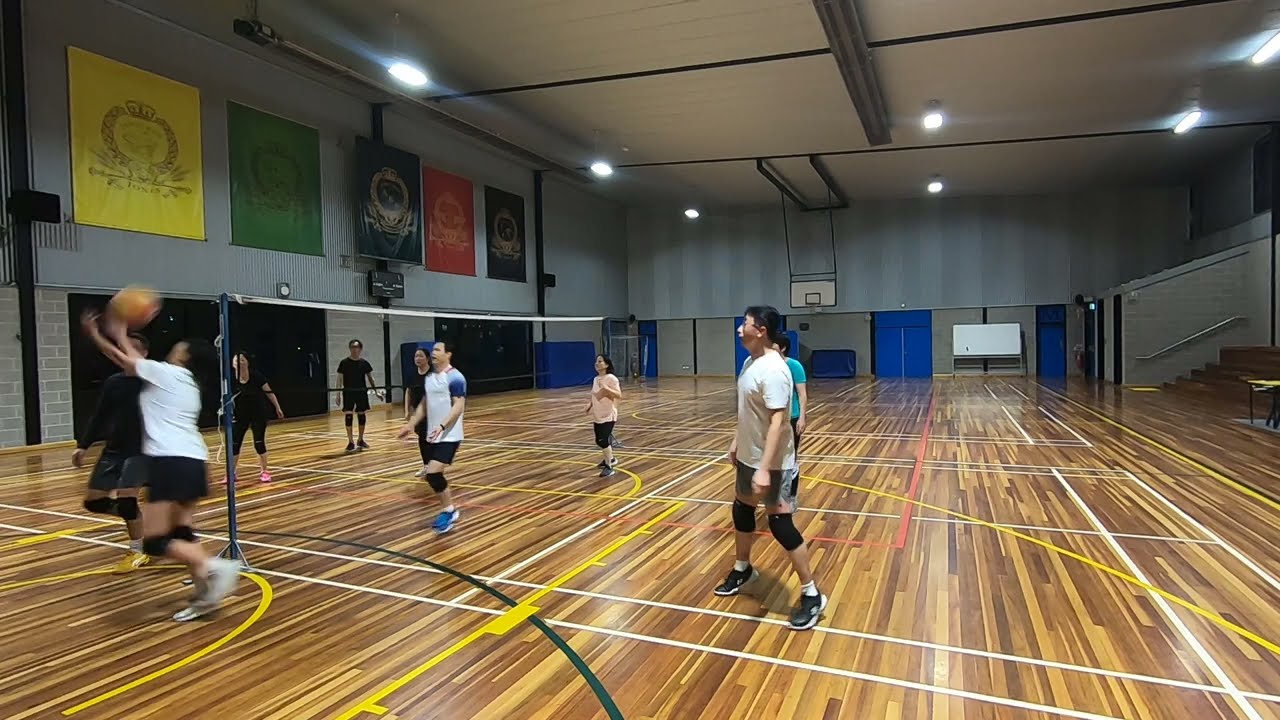In the image, we see a lively scene inside a gymnasium where people are engaged in a spirited game of volleyball. The gym's floor is made of wooden planks arranged in a striped pattern, with different shades of brown. Several players are in the midst of the action, with a bright orange ball seen in mid-air on the left side, just above the net that separates the two teams. The team on the left side of the net wears dark-colored t-shirts while the team on the right wears lighter ones. The players appear to be adults in their 30s, and it's a mixed team of men and women, predominantly of Asian descent.

The gymnasium itself is well-lit by ceiling lights, as there seems to be no natural light—suggesting it's evening or that the gym lacks windows. The ceiling is not very high, adding to the cozy, indoor feel. On the right, there are blue doors and bleachers, while the back wall on the left is black and appears to be cinder block with banners hanging above. The court features painted lines and a few flags hanging from the walls, giving the setting a sense of school spirit or community involvement. The overall ambiance hints at a friendly, competitive game taking place in a community or school setting under artificial lighting.